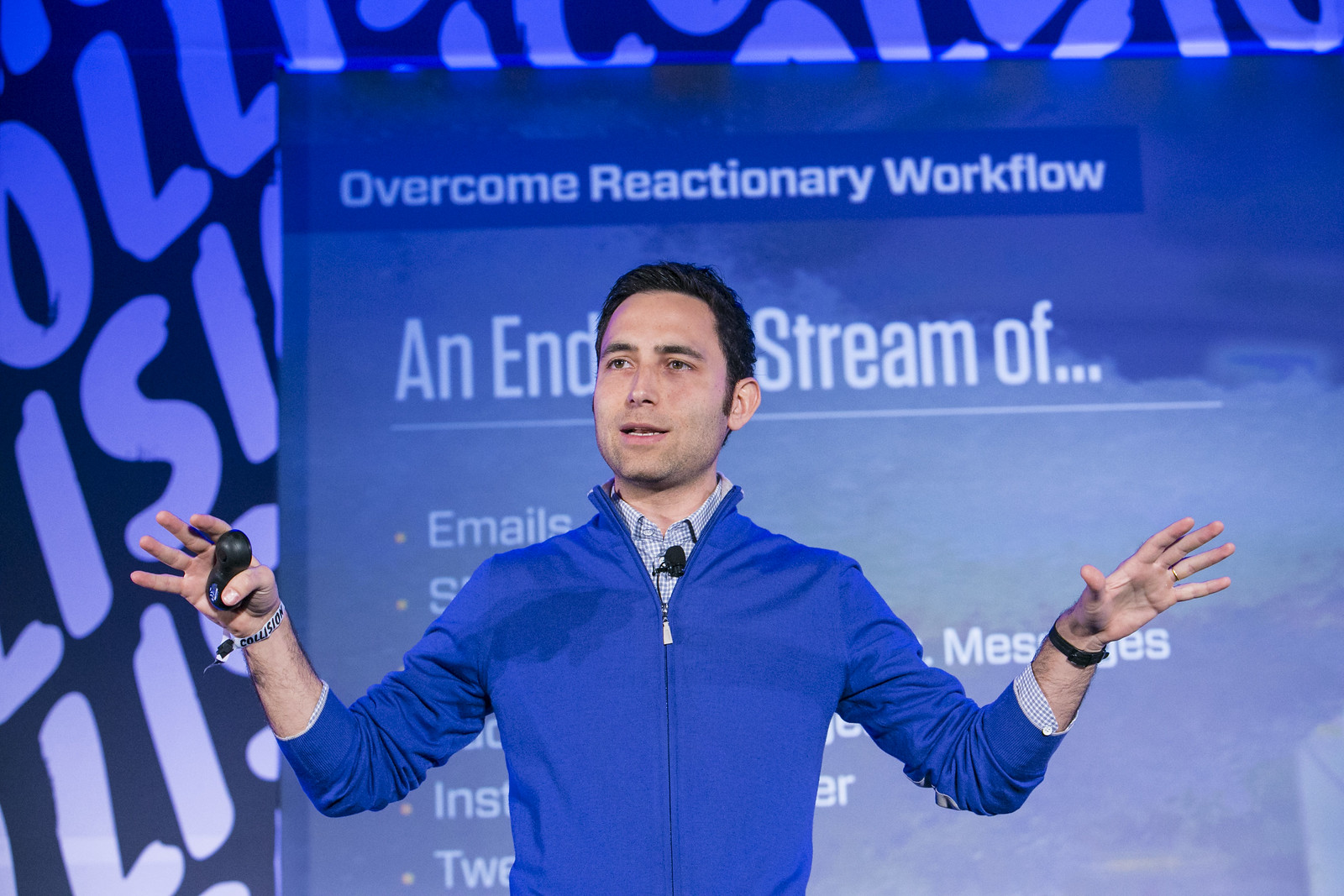In this wide rectangular image, a man with light skin and dark brown hair is giving a presentation, visible from the torso up. He is dressed in a white and blue checkered collared shirt beneath a bright blue zip-up long-sleeve top. His posture shows both arms raised and bent at the elbows, with a black remote in his left hand, adorned with a COLLISION wristband. On his right wrist, he wears a watch, and a ring is visible on one of his fingers. A microphone is clipped to his clothing. The man slightly looks to the left, while behind him, a blue PowerPoint slide is displayed, featuring the words "OVERCOME REACTIONARY WORKLOAD" in white over a dark blue rectangle at the top, with fragments of text to his left and right reading "an end" and "stream of..." respectively. The background of the slide is light blue with some cloud designs.